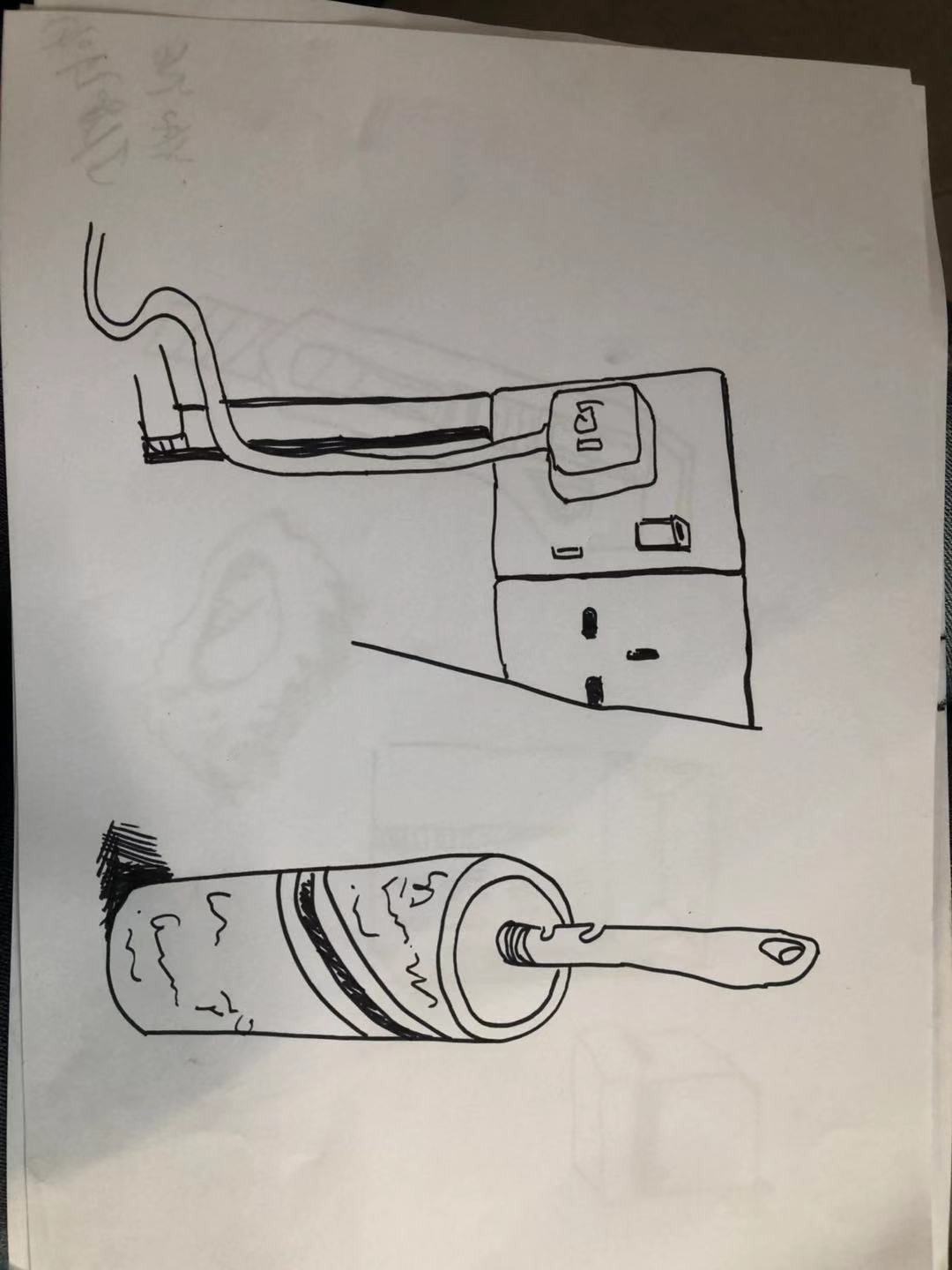A minimalist, black pen illustration on white paper depicts a double electrical outlet and a lint roller. The artwork features a sketch-style outline with clean, simple lines. The double outlet includes one open socket, providing a clear view of its interior. The opposite socket is occupied by a cube-shaped plug, from which a cord extends downward along the imagined wall. Adjacent to the outlet, the lint roller is rendered as a cylindrical shape, complete with a distinguishing stripe around its label. A small hole is illustrated at the top of the lint roller's handle, adding a touch of authenticity to the depiction.